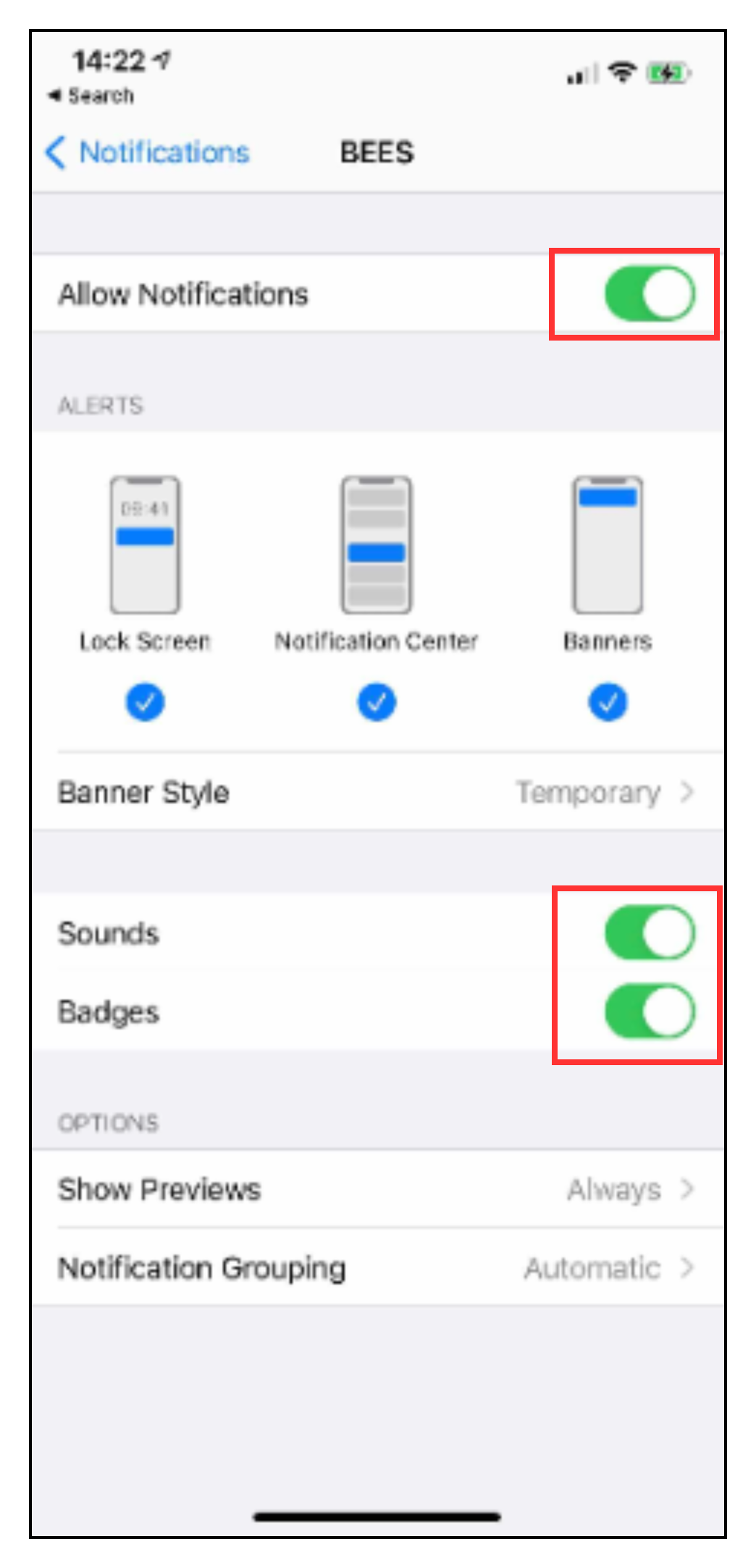The image depicts a cell phone screen displaying a settings interface. At the top-left corner, there's a time displayed as "14:22", and on the top-right corner, there are indicators for cellular signal strength, Wi-Fi connection, and data usage. The battery icon shows that the battery is charging, appearing mostly green.

Below the status bar, there's a search bar on the left side, displayed in black, and adjacent to it, there's a blue "Notifications" label accompanied by a left-facing arrow. Centered below this is the capitalized letter "B".

A grey band separates this section from the main content. The primary background here is white, featuring a toggle labeled "Allow Notifications" which is switched on, indicated by a red check mark.

Further down, on a grey background, there's a section titled "Alerts" displaying three screenshots representing different alert options: "Lock Screen" (checked with blue), "Notification Center" (highlighted and checked with blue), and "Banners" (also checked with blue). The banner style is set to "Temporary," indicated by a right-facing arrow.

Below the "Alerts" section, under "Sounds and Badges," both options are toggled on and appear green, highlighted by a red box. The "Options" section is next, where "Show Previews" is set to "Always," directed by a right-facing arrow. Below that, "Notification Grouping" is set to "Automatic," followed by another right-facing arrow.

At the bottom of the screen, a black line appears, running across the middle. The highlighted elements like "Allow Notifications," "Sounds," and "Badges," each boxed in red, imply this screen could be part of an educational tool, emphasizing the importance of setting notification preferences.